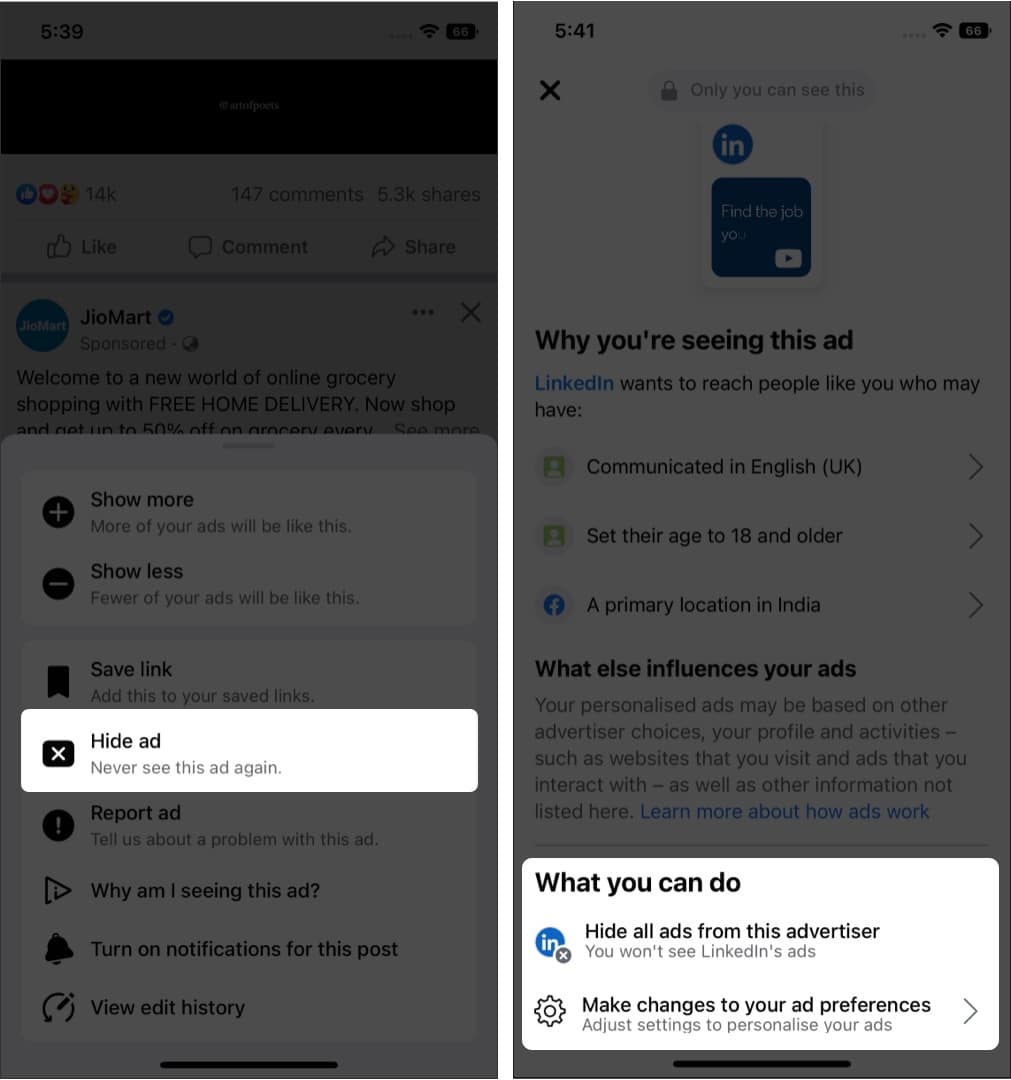In this composite image, which consists of two juxtaposed screenshots, the left screenshot is captured from Facebook. It illustrates an interaction with an advertisement, where the user has clicked on an icon to expand the ad options. Notably, the image has been photoshopped to emphasize the "Hide ad" button by highlighting it, while the rest of the options, such as "Show more," "Save link," "Report ad," "Why am I seeing this ad," and "Turn on notifications for this post," are shaded in dark gray. The advertisement is from Geomart, clearly marked as sponsored content.

The screenshot on the right appears to be from the same iPhone, indicated by the home bar at the bottom. This page delves into the reasons why the user is seeing the specific ad, explaining that LinkedIn wants to reach individuals who have communicated in English (UK), are aged 18 or older, and primarily located in India. It further elaborates that the personalization of ads may be influenced by other advertisers' choices, the user’s profile, activities, visited websites, and previously interacted with ads. Highlighted at the bottom of this screenshot are options for user action, such as "Hide all ads" and "Make changes to your ad preferences."

This detailed dual-screen capture renders a comprehensive visual narrative of ad targeting and user interaction on social media platforms.